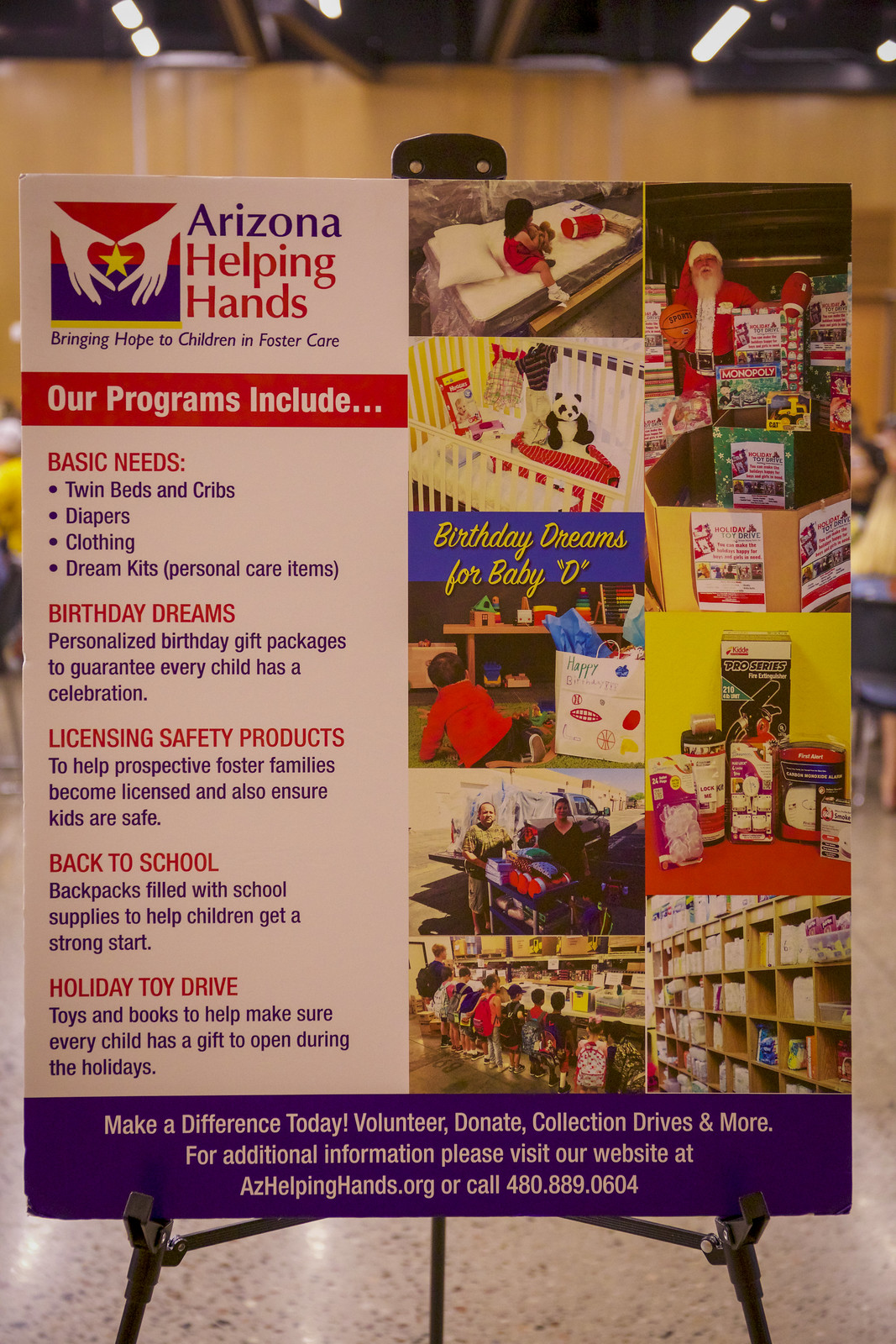The image depicts a large promotional board display for Arizona Helping Hands, positioned on a stand. The exact material of the stand is unclear, but it features visible legs extending below the board and a support structure rising from the middle top. The board is split into two main sections. On the left side, there is a detailed list of the organization's programs beneath an emblem with the title "Arizona Helping Hands," accompanied by a slogan, "Bringing hope to children in foster care." Below this, a red band labeled "Our Programs Include" introduces various initiatives:

- "Basic Needs" with details like twin beds, cribs, diapers, clothing, and personal care items.
- "Birthday Dreams," offering personalized birthday gift packages.
- "Licensing Safety Products," assisting prospective foster families with licensing and ensuring safety.
- "Back to School," providing backpacks filled with school supplies.
- "Holiday Toy Drive," ensuring every child has a gift during the holidays.

The right side of the board showcases two columns of images including scenes of children, a Santa Claus, shelves filled with toys, and a girl in a crib surrounded by toys. Among the images, there's a blue rectangle that partially reads "Birthday Dreams for Baby," and various images related to their projects, such as toiletries and bedding supplies.

A purple border at the bottom includes white text urging people to "Make a difference today" through volunteering, donations, and collection drives. Additional contact information is provided: "For additional info, please visit our website at azhelpinghands.org or call 480-889-0604."